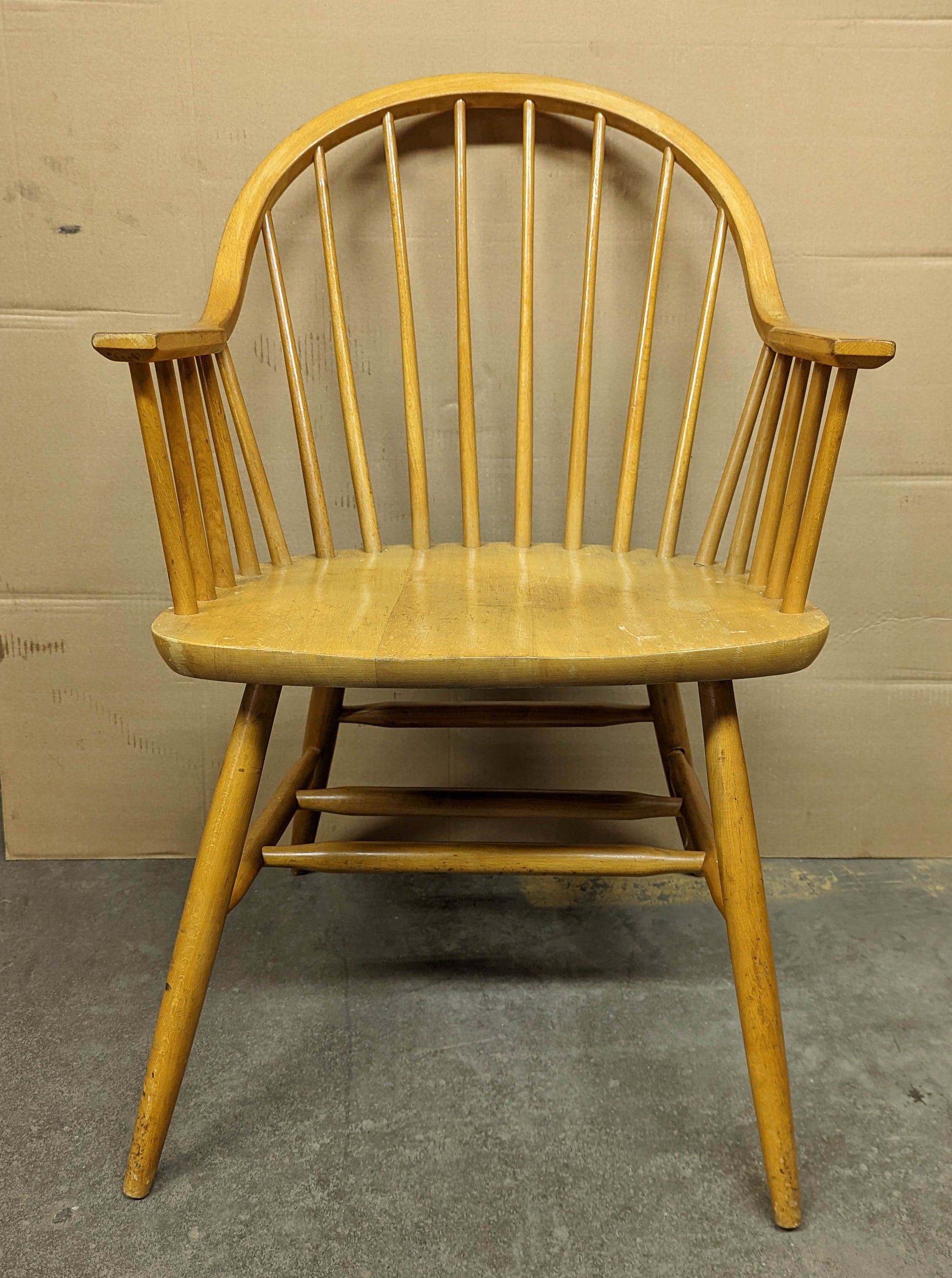The image features an old, wooden chair with a distinctive design reminiscent of the 1960s or 70s. The chair is characterized by a rounded, arched back composed of numerous wooden dowels—eight arranged vertically at the back and four on each side. The dowels are anchored by a top piece of wood that creates a unified, sturdy arch. The seat of the chair is flat and plain, supported by four wooden legs. These legs are interconnected horizontally with similar wooden dowels, adding to the chair's stability. The wood has a light tan, yellowish hue, and the chair shows signs of aging and wear, including scuffs near the feet. Surrounding the chair is a room with a tan-painted concrete wall marred by black scuffs. The speckled gray floor, presumably cement, has paint splatters likely from a hasty wall painting job. The background also includes beige rectangular pavers, adding texture to the setting.